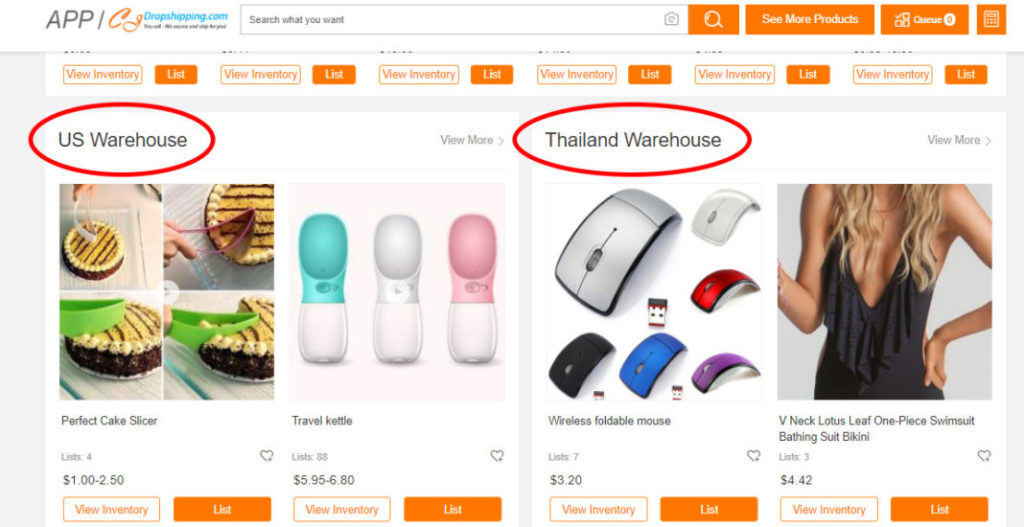The image depicts a section of the CJ Dropshipping website. 

At the top left, the word "App" is displayed in gray text. To the right of it, "CJ Dropshipping.com" is written, with "CJ" in orange and "Dropshipping.com" in blue. Adjacent to this is a search bar containing the placeholder text "Search what you want". In the top right corner, there are three orange buttons labeled "See More Product," "Queue," and an icon of a calculator.

Beneath this section, an inventory list is visible. The phrase "Your Inventory" is highlighted in orange, as is the word "List." The inventory is organized into four products, divided into two sections of two products each.

On the left side, the section is labeled "US Warehouse" in black text, outlined in a red rectangle, indicating these products are stored in a US warehouse. The first product featured is a Perfect Cake Slicer, which is green, white, and red, priced between $1.00 and $2.50. Below the product are two buttons: "Your Inventory" in white and "List" in orange. The second product in the US warehouse section is a Travel Kettle, priced between $5.95 and $6.80.

On the right side, the section is marked "Thailand Warehouse," also outlined in red. The first product here is a Wireless Foldable Mouse, available in various colors including gray, black, blue, pink, purple, red, and silver, priced at $3.20. The final product listed is a V-Neck Lotus Leaf One-Piece Swimsuit, priced at $4.42.

Each product entry includes the same two buttons for inventory management: "Your Inventory" in white and "List" in orange.